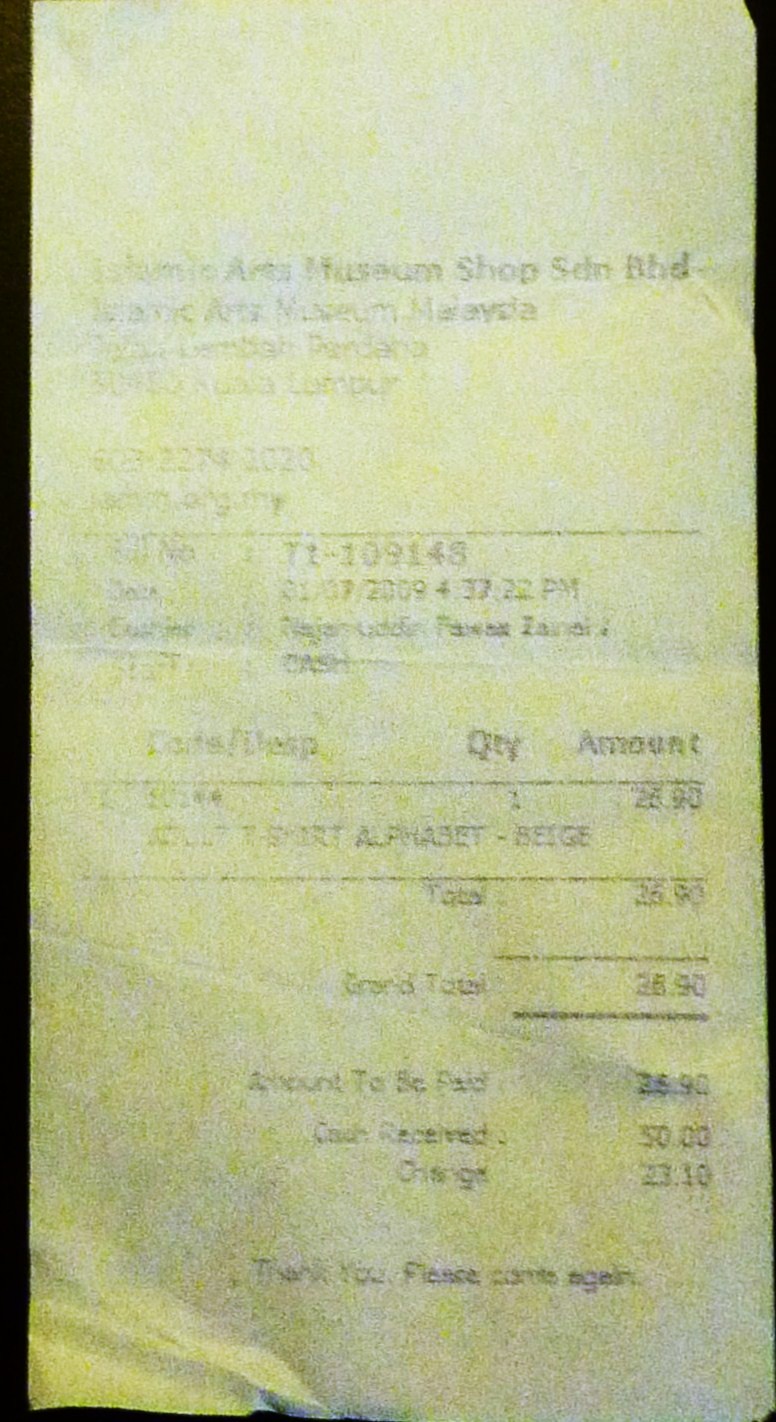The photograph depicts a damaged and somewhat faded receipt from the Islamic Arts Museum Shop, located on Sedan Boulevard, Malaysia. The receipt has a yellowish tinge, particularly noticeable at the top where the shop's name and address are partially obscured but still legible. Moving further down, a date is faintly visible, along with a transaction detail showing the purchase of a single item priced at $26.90. The total amount paid was $26.90, indicating no tax was applied. The receipt also notes that the customer paid with $50 and received $23.10 in change. At the bottom of the receipt, a courteous message reads, "Thank you, please come again."